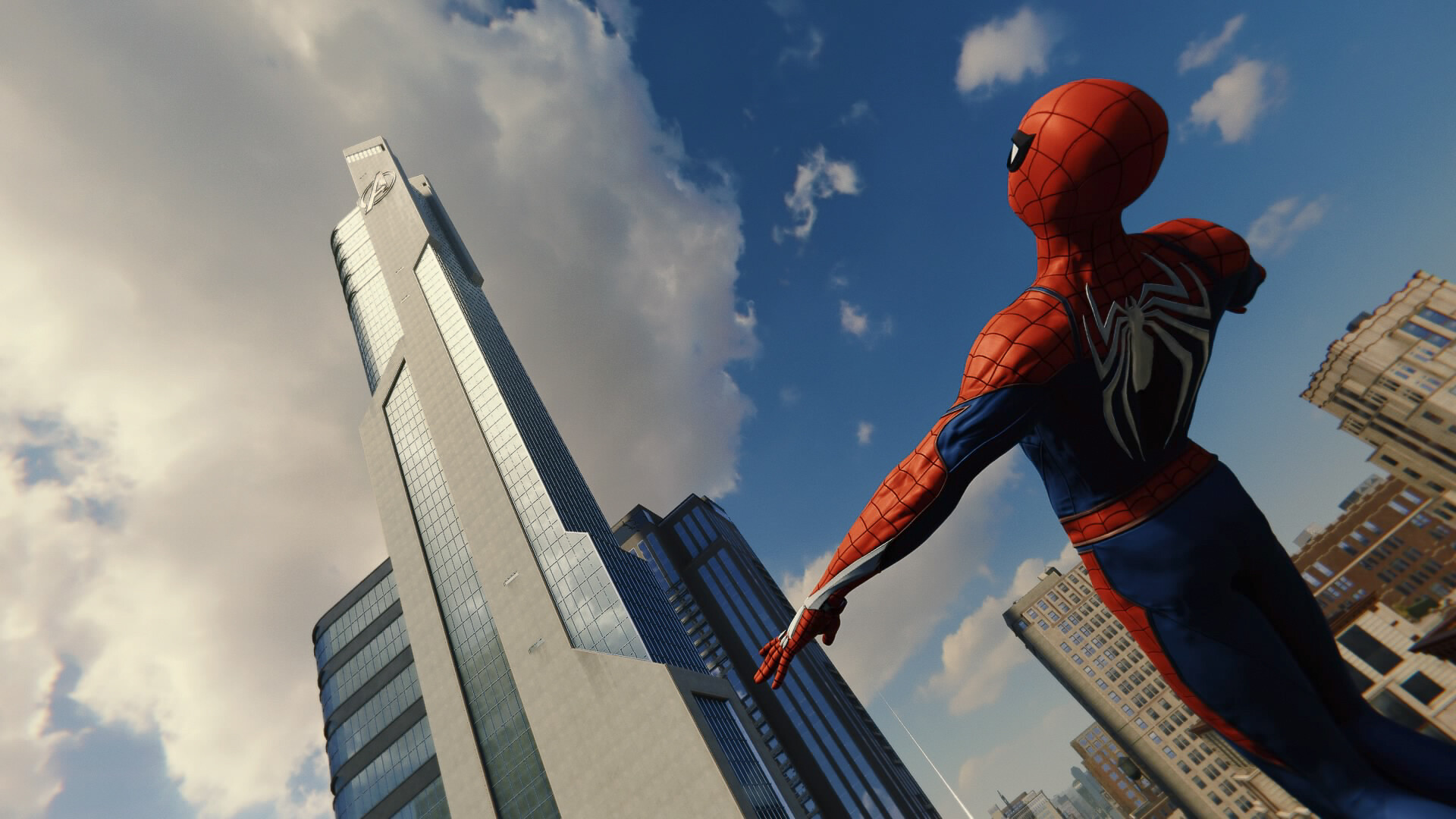The image depicts a computer-generated scene from a Spider-Man movie, featuring Spider-Man in a detailed red and blue bodysuit with a prominent white spider emblem on his back. The character is clearly rendered with CGI, emphasizing his intricate costume details: red fabric covering his head and shoulders, red extending partially down his arms, blue pants, and white areas around the eyes outlined in blue. Spider-Man is shown falling backward from a concrete and glass skyscraper, which is angled to the left and features a tall tower and shorter glass sections. His head is directed towards the top right of the image, while his legs extend towards the bottom right, arms spread outwards at his sides. The bright blue sky with large, fluffy white clouds dominates the background. Additional city buildings of varying heights are visible in the distance, enhancing the metropolitan ambiance of the scene.